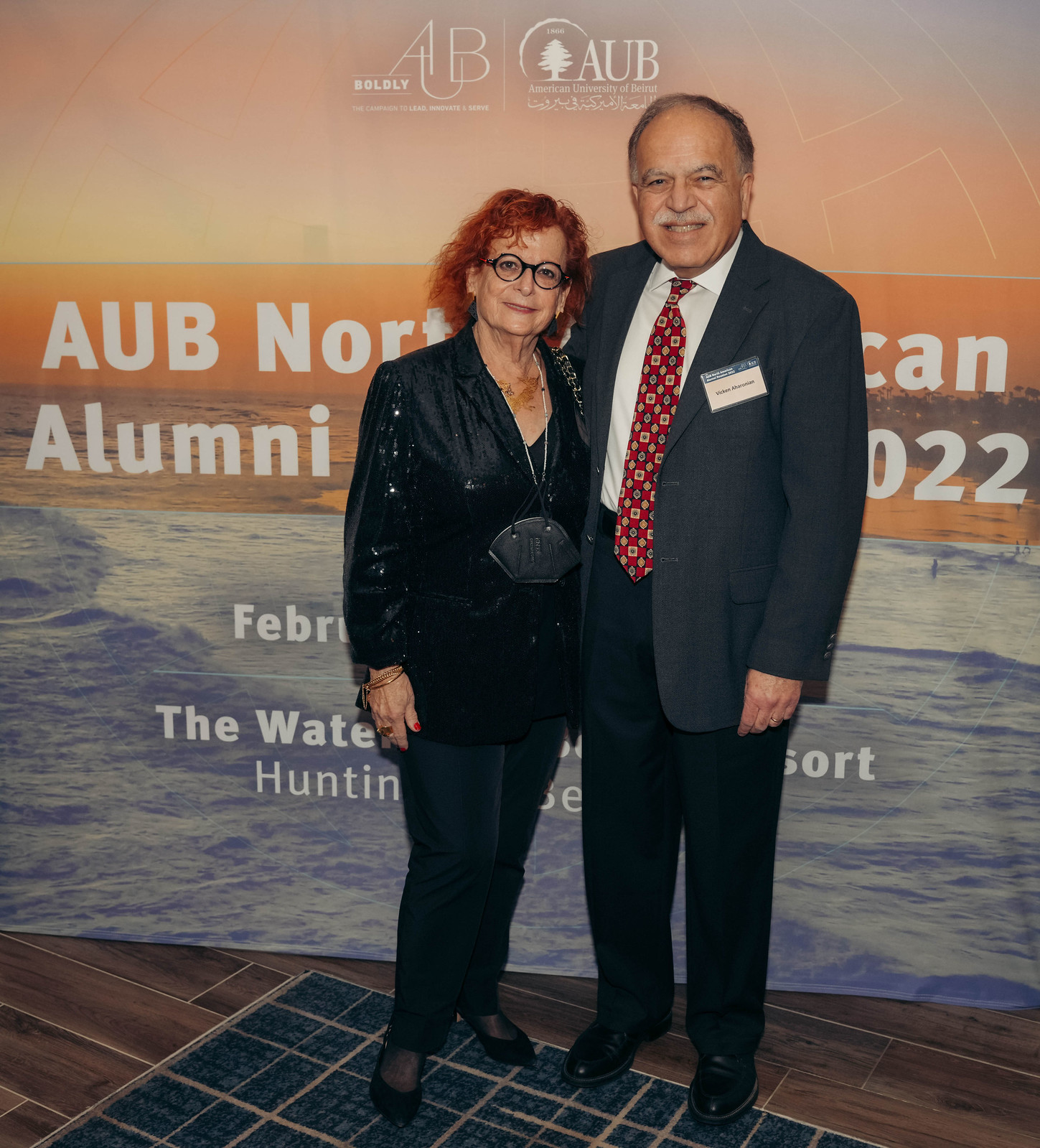In this image, two individuals are posing for a photo at what appears to be an alumni event for the American University of Beirut. They are standing on a brown and blue wooden floor with a back wall that features a design resembling an ocean, beach shoreline, and sunset sky in blue, orange, and white hues. Bold text on the banner behind them reads "AUB, AUB, American University of Beirut, AUB alumni," with some words and numbers partially obscured by their bodies, indicating a date in February and the year '22.

The person on the right is a man with a white complexion, wearing a navy suit jacket and pants, white shirt, and a checkered tie in shades of red, blue, yellow, and black. He has a gray mustache and wears black shoes. The woman on the left has red hair, wears black glasses, and is dressed in an all-black outfit with long sleeves. She accessorizes with necklaces, bracelets, and a pouch or name tag attached to her chest. Both individuals are smiling and have their arms around each other’s shoulders, with the man’s arm around the woman's shoulder, capturing a moment of camaraderie at the event.